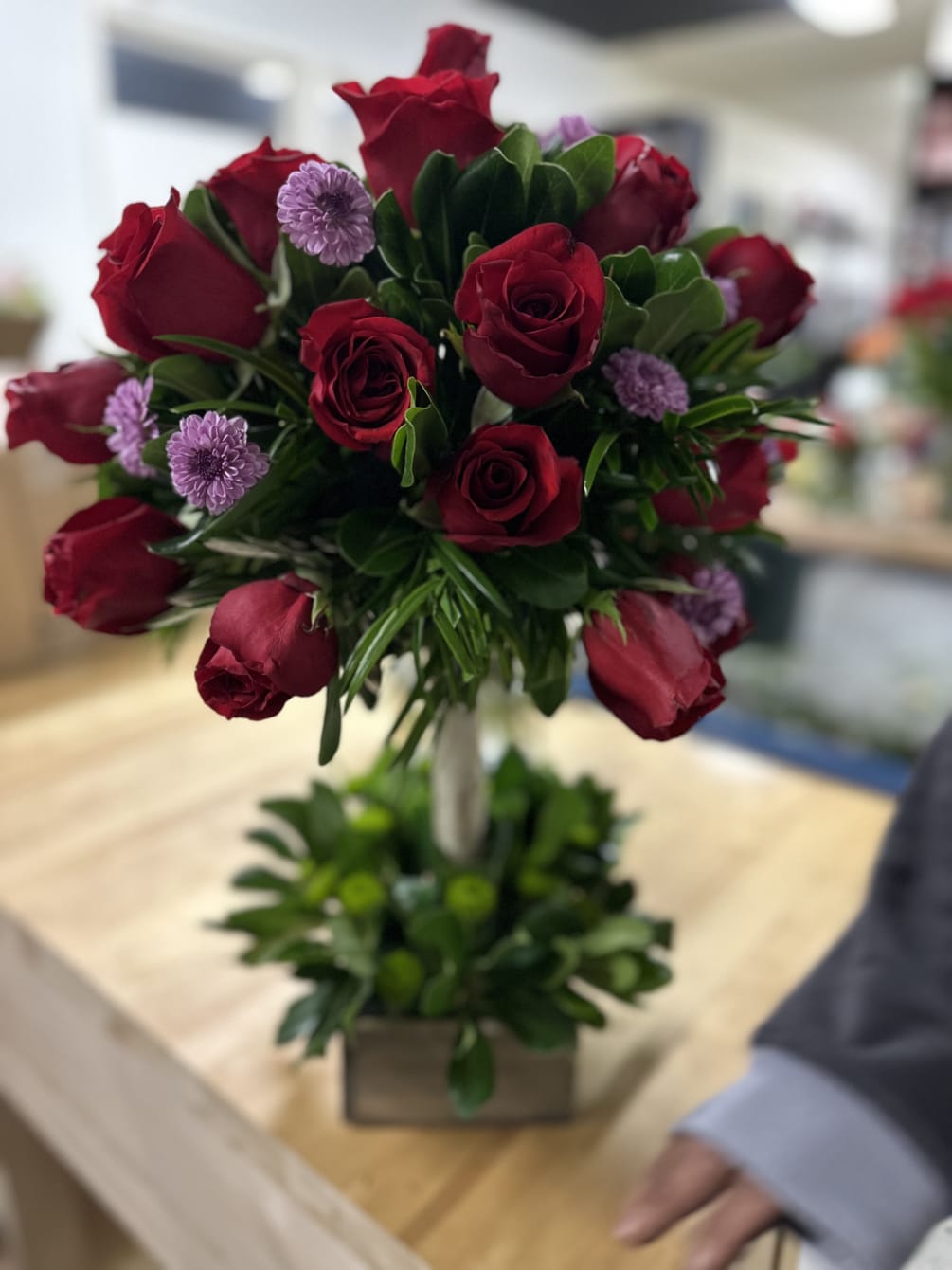This detailed photo captures an intricately arranged floral centerpiece situated on a light wood grain table or desk in an office or public space. The base of the centerpiece is a gold, square box, partly visible, from which lush, thick dark green foliage emerges. A white or cream-colored pole rises from the greenery, leading to the main floral display. The centerpiece features an abundance of red roses, coupled with purple chrysanthemums, beautifully accentuated by the same type of dark green leaves. In the bottom right corner of the image, the arm of a person wearing a navy jacket is visible, with two or three fingers extending into the frame. The person's presence adds a subtle human element to the otherwise aesthetic arrangement. The overall setting is subtly elegant, highlighting the thoughtful combination of colors and textures in the floral arrangement.